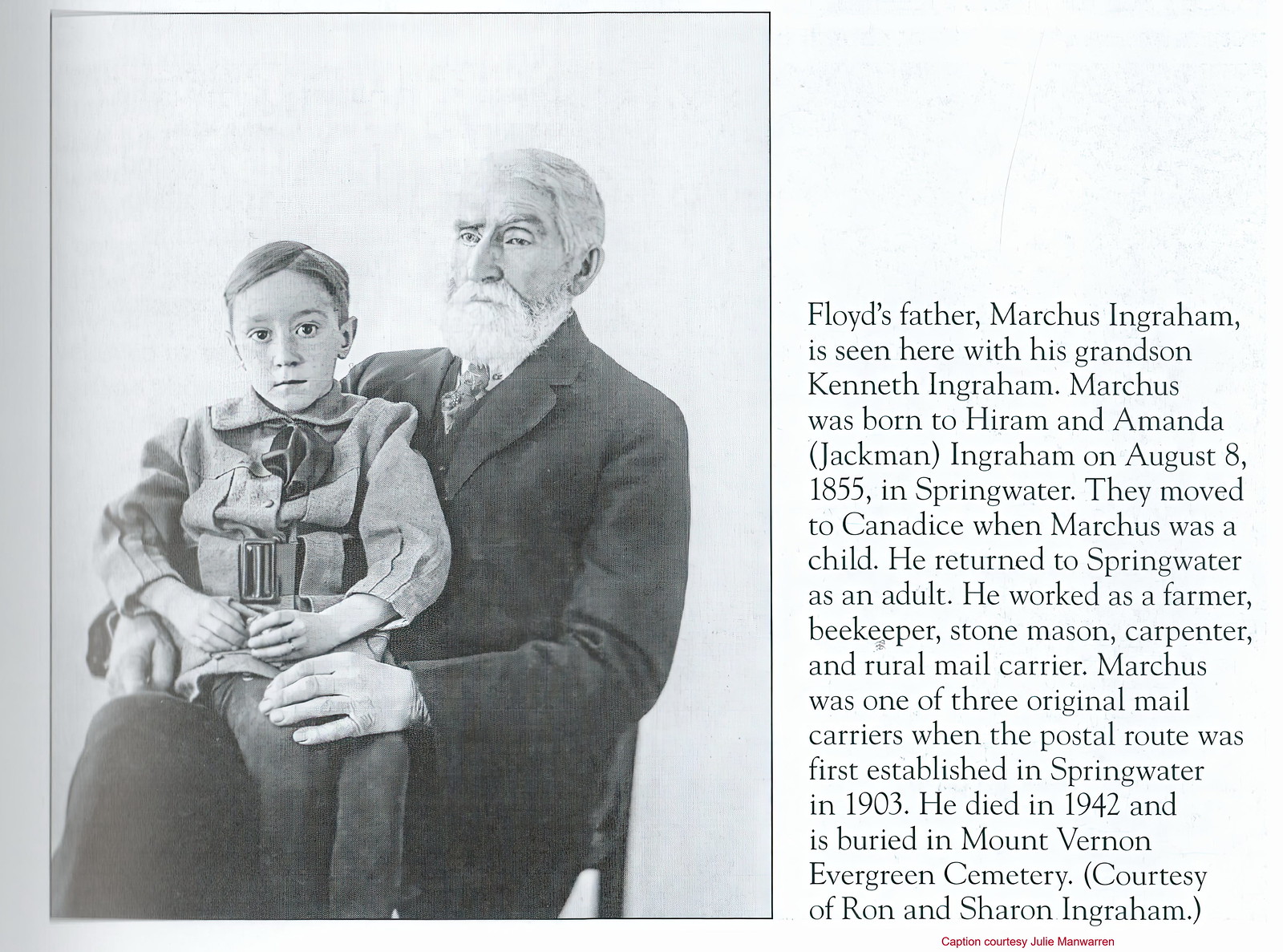The image appears to be a scanned page from a book, featuring a black-and-white photograph on the left-hand side and descriptive text on the right. The photograph captures an older gentleman, Marcus Ingram, seated formally in a dark suit complete with a vest, tie, and white shirt. His hair is neatly groomed, and he sits with one leg crossed over the other. On his lap sits his young grandson, Kenneth Ingram, who appears to be around six or seven years old. Kenneth is also dressed for the occasion, wearing a formal coat with a large belt and an early 20th-century style tie. Both subjects are looking directly at the camera with serious expressions.

The accompanying text on the right provides a detailed background on Marcus Ingram, stating that he was born to Haram and Amanda Jackman Ingram on August 8, 1855, in Springwater. Marcus's family relocated to Kansas during his childhood, but he eventually returned to Springwater as an adult. Throughout his life, Marcus worked in various professions including as a farmer, beekeeper, stonemason, carpenter, and rural mail carrier. Notably, Marcus was one of the three original mail carriers when the Postal Route was first established in Springwater in 1903. He passed away in 1942 and is interred at Mount Vernon Evergreen Cemetery.